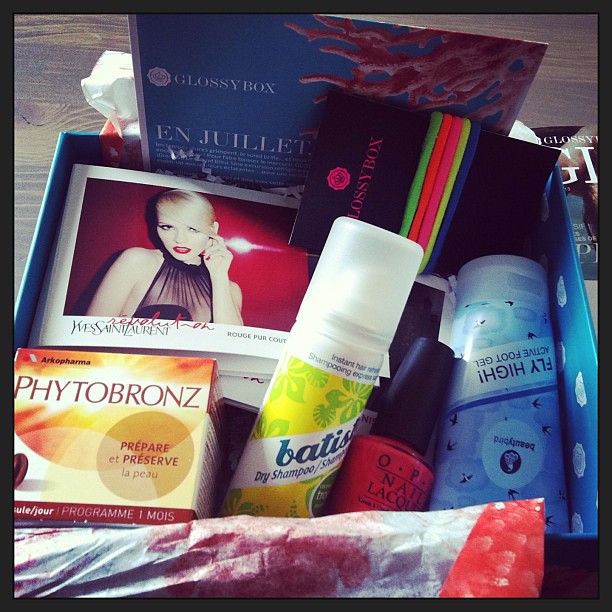In this image, a variety of beauty and personal care products are displayed on a brown wooden surface, appearing to occupy the entire frame. Central among the items is a yellow and white bottle of dry shampoo, an orange-red nail polish from OPI, and a lavender-colored tube of Fly High Active Foot Gel. Also present are some bright, fluorescent hair bands wrapped around a black piece of paper, and a white box with red and orange accents labeled PhytoBronze. The collection is organized within an open blue shoebox. Additionally, there are unmarked bottles and tissue paper in white and red colors, scattered around. A picture of a model with blonde hair posing against a red background is also visible, adding to the eclectic mix of items. This indoor setting appears to be someone's organized display or collection of beauty products, showcasing various colors like black, brown, blue, pink, red, orange, yellow, green, lime green, and purple.